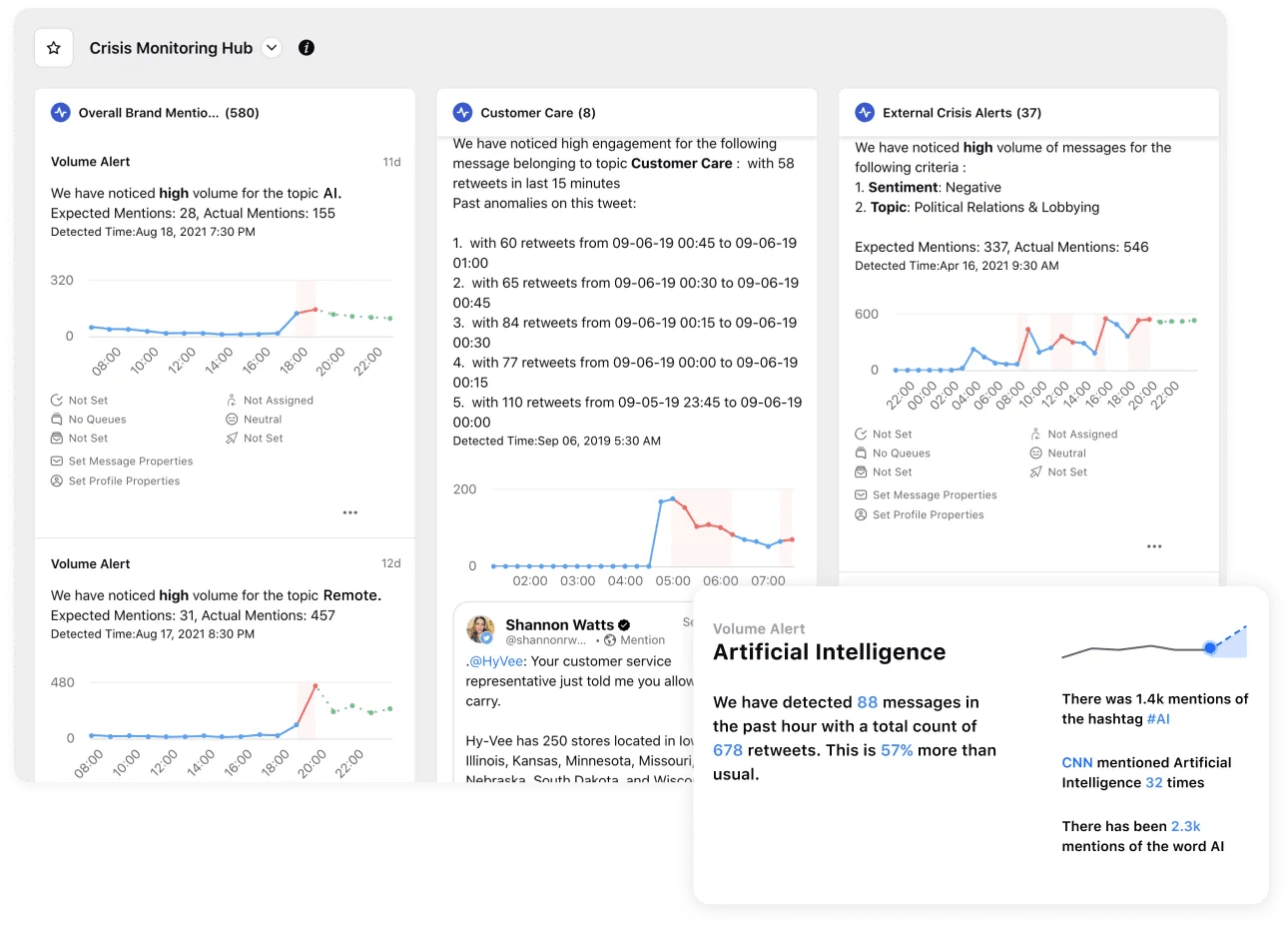**Detailed Caption:**

In the image, there is a prominent pop-up window located on the right-hand side of the screen. The pop-up window features a rectangular shape, with its upper left-hand corner shaded in gray. This gray section contains the text "Volume Alert" in black. Below it, the text "Artificial Intelligence" is also displayed in black, followed by the message, "We have detected 88 messages in the past hour," where the number of messages, "88," is highlighted in blue. Additionally, the pop-up states, "A total count of 678 retweets," with "678 retweets" again highlighted in blue. It notes a 57% increase, which is colored in blue as well.

Next to this section, it reads, "There was 1.4 mentions of the hashtag," with "#AI" highlighted in blue. It also mentions "CNN," marked in blue, followed by, "mentioned artificial intelligence," with "32 times" highlighted in blue. Furthermore, it reports, "There has been 2.3K measures of the word AI," where "2.3K measures" is highlighted in blue.

The background of the main page is gray. In the top left-hand corner, it states "Crisis Management Hub" in black text. In the first column, it reads "Overall Brand Mentioning," with parentheses noting "580 volume alert." The message continues to explain that there has been a high volume of the topic "AI," with expected mentions at 28 and actual mentions at 155, detected on August 18, 2021, at 7 p.m.

Subsequently, it highlights a high value detected for the topic "remote," with expected mentions at 31 and actual mentions at 457, detected on August 17, 2021, at 8:30 p.m. Under the section "Customer Care," it indicates high engagement within the last 15 minutes for messages related to "AI," noting 58 retweets.

Finally, it displays an "External Crisis Alert," identifying a significant volume of messages related to negative sentiments on political relations and lobbying. The expected mentions were at 337, with actual mentions rising to 546, detected on April 16, 2021, at 9:30 a.m.